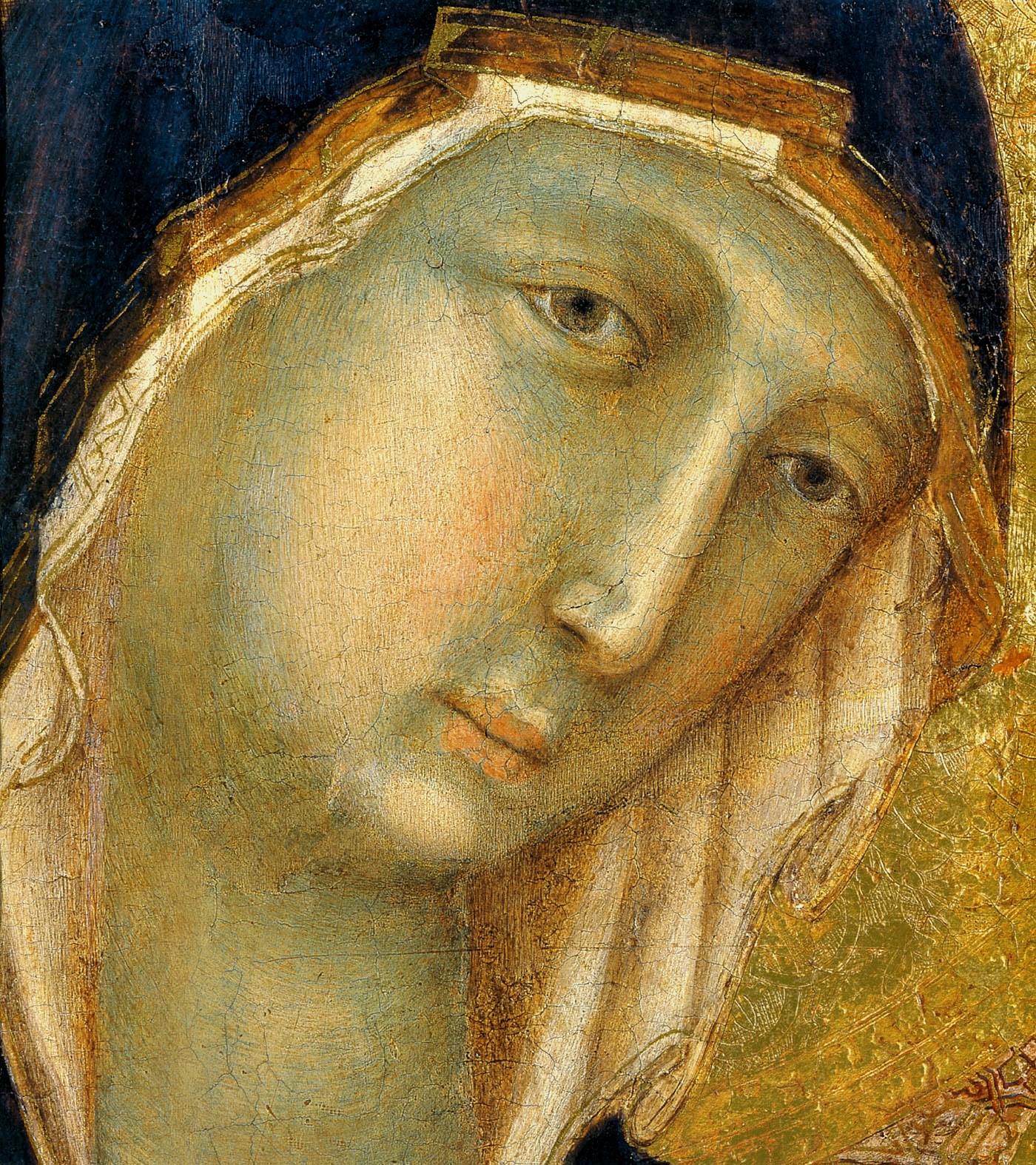This image captures a photograph of a very old painting that exhibits significant signs of aging and wear. The subject is a woman, likely a nun or a holy figure, who is gazing to the left with a slightly sad expression. Her features include a long nose, pursed lips, and a strong neck. She wears a distinctive headdress with a white bottom, orange middle section, and blue top, adorned with a border of gold. The technique used by the original artist is evident as chipping in the outer layers of paint reveals the underlying green base layer, a common practice of the time to build up flesh tones. The paint surface shows extensive cracking, attesting to the painting's age. Intricate gold flake gilded elements with fine knotwork adorn the lower right-hand side of the painting and remain remarkably intact for the artwork's age. Notably, this piece lacks a visible signature.